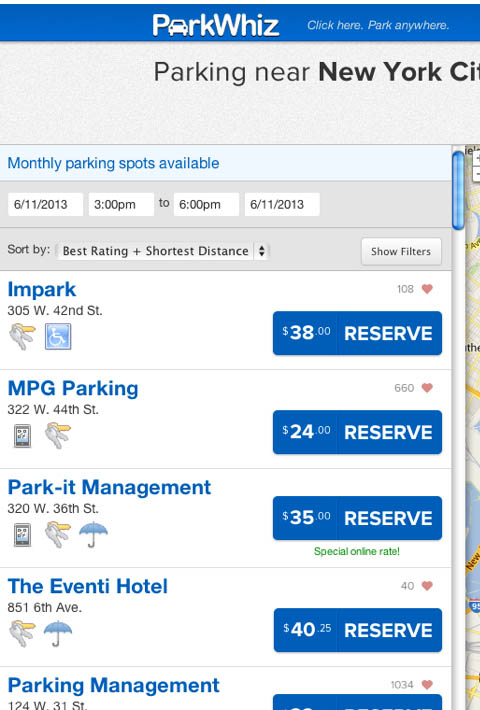The image depicts a screen capture of a section of a webpage designed for booking parking spots. The webpage features a clean, white background with blue accents, including blue text and buttons. At the top of the page is a blue navigation bar with white text that reads, "Pack With." Directly below, another blue header reads "Packing Near New York." 

Underneath this header, light blue text on a blue background states, "Monthly Packing Spots Available." Further down, time slots are listed on white rectangular buttons.

The main content showcases several rows of available parking spots. In the first row, blue text indicates "Impact," with smaller black text providing the address "305 West 42nd Street." An icon of keys and a handicap symbol is also visible. To the right of this listing, there is a blue button labeled "$38 Reserve."